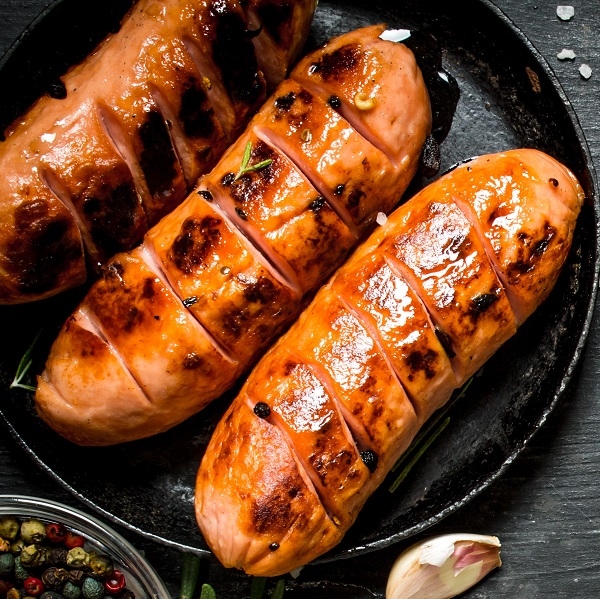The image showcases a close-up of three pinkish sausage links with black char marks, sizzling in a cast iron skillet. Each sausage has about five or six cuts across and is garnished with a small green herb and flecks of salt. The sausage link at the top features the most prominent char marks. To the bottom of the skillet, part of a glass bowl filled with multicolored peppercorns in shades of green, red, and blue is visible. To the right of the skillet lies an unpeeled clove of garlic, white with hints of pink. The top right section of the image contains scattered white sea salt flakes, adding to the texture and flavor of the scene.